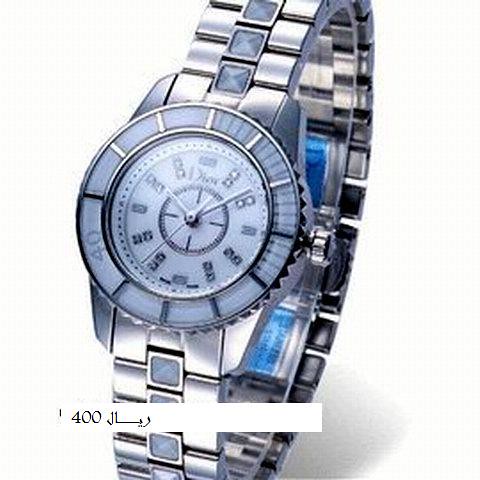In this vertically-oriented rectangular image, we see a digitally enhanced photograph of a men's wristwatch. The watch's band is robust and designed with three interwoven rows of silver, creating a stretchy bracelet-style strap that can be slipped over the hand with ease. The watch face features a silver and white color palette. Around the dial, inscrutable black markings, which resemble a hybrid of numbers and alphabetical symbols, are displayed, giving the impression of number eights rather than distinct numerals. The time appears to be set at 11:10. Overlaid on the watch face is bold, white text that reads "400," providing a striking contrast to the watch's silver and white tones.